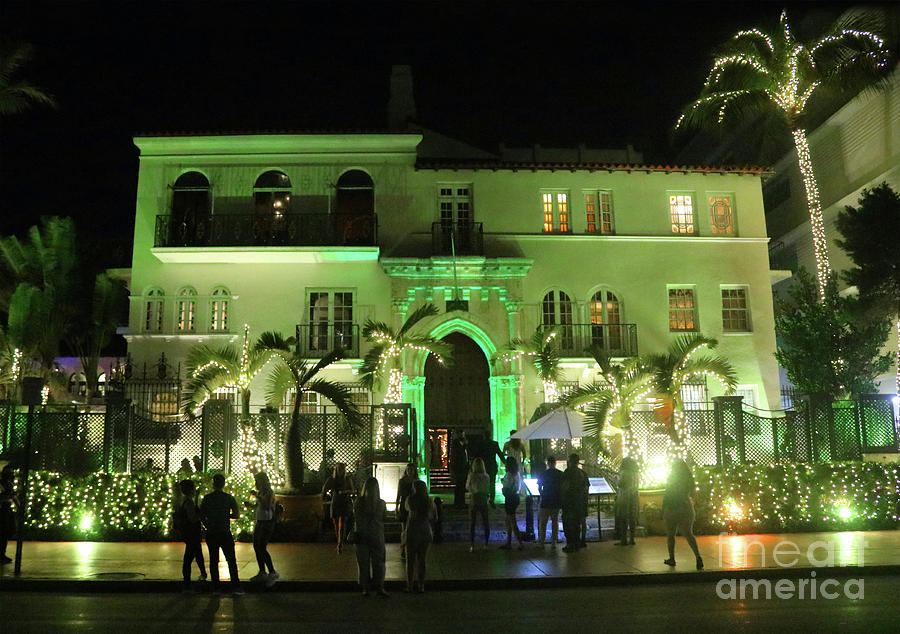The image depicts a nighttime street view of a large, multi-storied house that gives off the impression of a hotel. The scene features a dark, black sky, and the house is prominently lit up with green accent lighting. The house is surrounded by a decorative fence, lined with hedges adorned with lights that flash in different colors. A large, rounded archway resembling a castle door, nearly two stories high, marks the entrance of the house.

In the foreground, there's a crowded sidewalk and road with approximately 20 people dressed in attire suitable for a night out or clubbing. Flanking the house are several palm trees wrapped in white, Christmas-like lights, creating a festive atmosphere. The right edge of the image includes a palm tree similarly decorated with white lights. The house has multiple balconies and all its windows are brightly lit, except for a few in the top left corner which remain dark.

Amid the illuminated bushes and hedges in front of the house, there's some transparent white lettering in the bottom right corner of the image that ambiguously reads "Fine Art America," adding a subtle artistic touch to the scene.